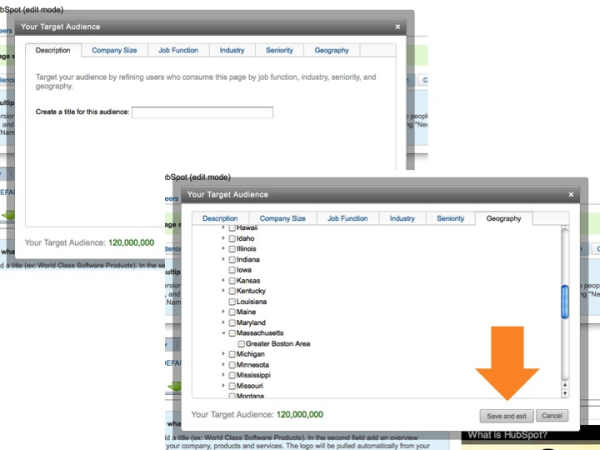This image features two overlapping screenshots of utility pages from the HubSpot software platform, commonly used for content marketing management. The two screenshots are arranged with one in the upper left corner and the other in the lower right corner.

The more prominent screenshot, positioned at the bottom right, showcases a header in gray with white font text that reads "Your Target Audience." Below the header, the background is white and displays a horizontal menu bar with options written in blue font: "Description," "Category Size," "Job Function," "Industry," "Seniority," and "Geography." The "Geography" tab is highlighted in gray, indicating it's the selected option. Below the menu, on the left side, the page lists U.S. states from Hawaii through Montana.

In the lower right corner of this screenshot, there is a large orange arrow directing attention to a button labeled "Save and Exit." On the left portion of the screen, the text "Your Target Audience, 120 million" is visible, indicating the scale of the audience being targeted.

In the upper left corner of the image, the second screenshot partially overlaps with the first. The overlapping design hints that these are administrative pages from HubSpot, as further suggested by a text rectangle at the bottom right of this screenshot with gray font on a black background that says, "What is HubSpot."

The detailed layout and the visible elements identify these images as part of the administrative pages used to manage and configure target audience settings within the HubSpot platform.